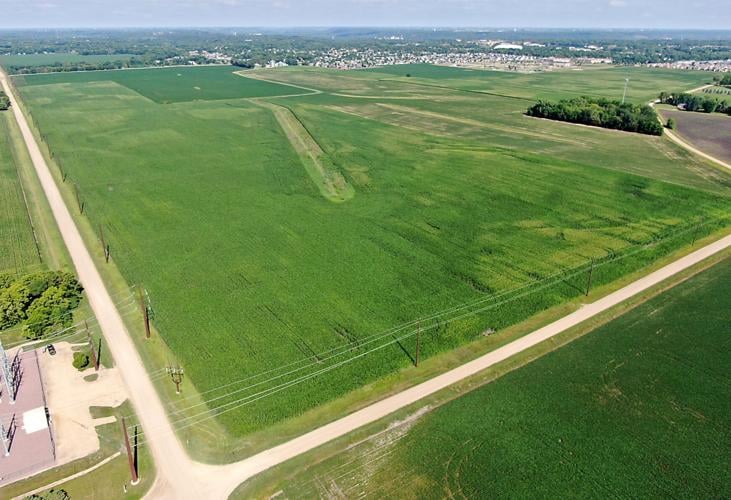The image is an aerial photograph, likely captured by a drone, showcasing a vast, flat green field. Dominating the left side of this expansive grassy landscape are two intersecting dirt roads, lined with rows of electrical poles and telephone wires. The different shades of green grasses add a rich texture to the field. In the far background, near the horizon, a cluster of small dots signifies a distant housing development or residential area. There's also a power station situated on the left, with lines extending out to the power poles. Patches of trees or bushes can be seen in the top right corner, next to a roadway that's partially visible at the edge of the photo. The sky above appears hazy, lending a soft focus to the distant elements of the image.